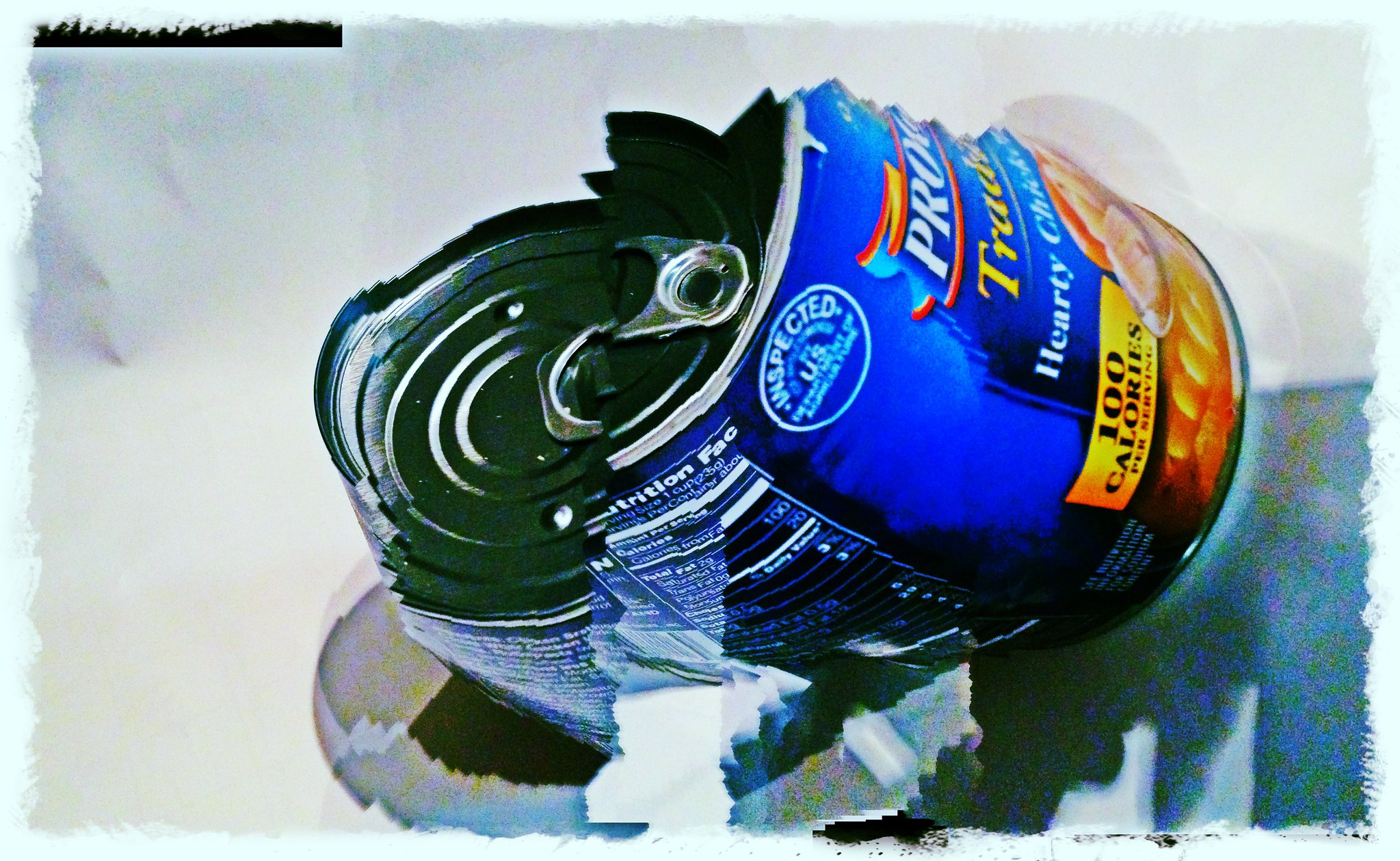The image presents an artistic depiction of a Progresso hearty chicken soup can, fragmented and reassembled in a visually striking manner. The can, which features a blue outer wrapping and a silver metal top with an easy-pull tab, appears distorted and cut up, with overlapping sections pasted in an eccentric, scrapbook-like fashion. Prominently displayed on the front is a picture of the soup, alongside a yellow rectangular text box that announces "100 calories per serving" in black text and the phrase "hearty chicken" in white text. The nutritional facts label, written in white text, is partially visible on the can's side. Set against a white wall and a blackish-gray table, the entire scene conveys a modern, slightly abstract artistic interpretation, almost as if the can has been dented or shattered, offering a unique and compelling visual experience.